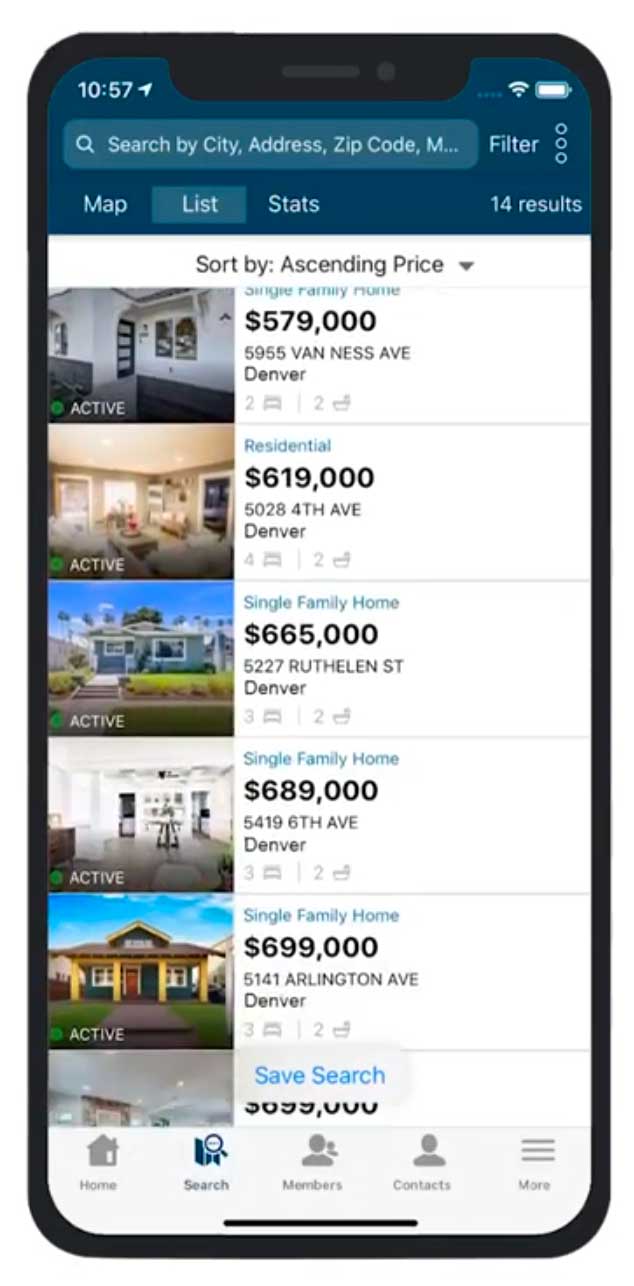Screenshot of a mobile phone display featuring a real estate search interface. At the top, the time is shown as 10:57 AM. The search bar includes options for searching by city, address, or zip code, and filters and views for map and list, with the list view currently selected. Statistics indicate 14 results, sorted by ascending price.

- The first listing shows a photograph of a white house labeled as a "Single Family Home," priced at $579,000, located at 5955 Van Ness Avenue, Denver. It has 2 bedrooms and 2 bathrooms.
- The second listing features a photo of a living room with predominantly white decor, labeled "Residential," priced at $619,000, located at 5028 4th Avenue, Denver. It offers 4 bedrooms and 2 bathrooms.
- The third listing presents an image of a single-story home in bluish-gray, labeled "Single Family Home," priced at $665,000, located at 5227 Ruthelen Street, Denver. It has 3 bedrooms and 2 bathrooms.
- The fourth listing includes a photograph of a white living room, labeled "Single Family Home," priced at $689,000, located at 5419 6th Avenue, Denver, featuring 3 bedrooms and 2 bathrooms.
- The final listing shows an image of a single-story home with four yellow pillars in the front, labeled "Single Family Home," priced at $699,000, located at 5141 Arlington Avenue, Denver. It includes 3 bedrooms and 2 bathrooms.

At the bottom of the interface, there is an option labeled "Safe search."